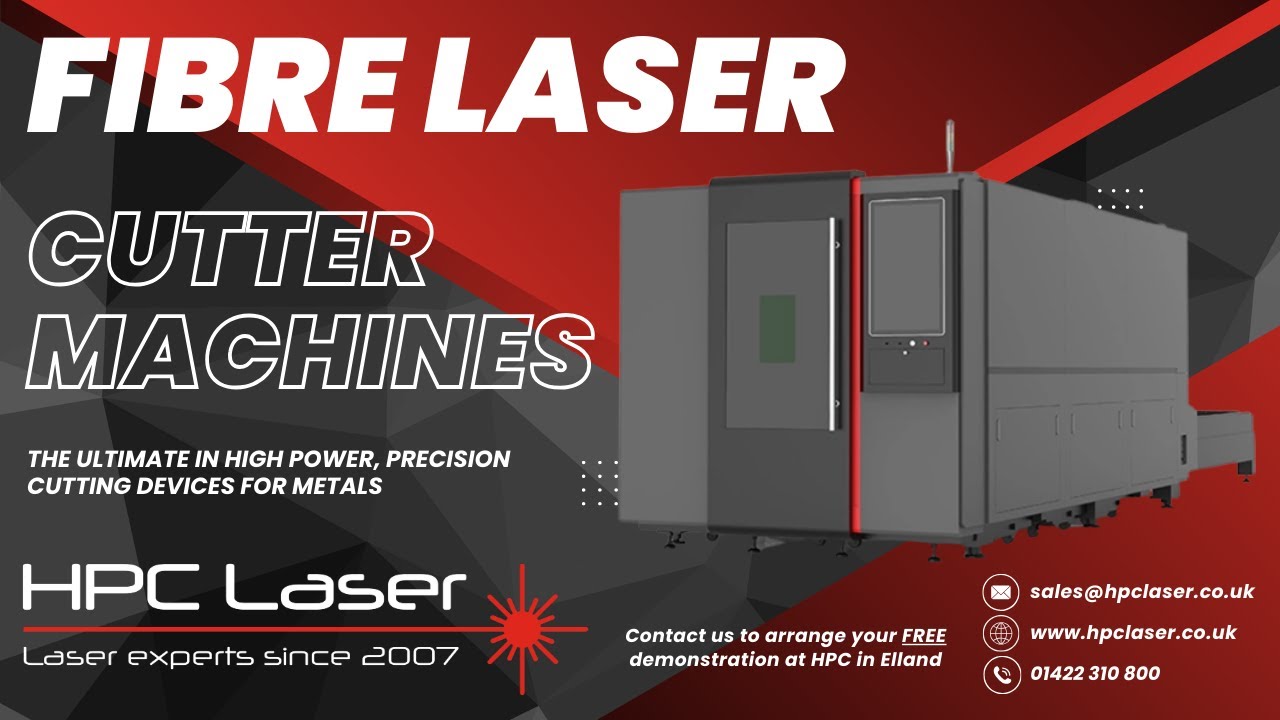The advertisement is a rectangular banner with a striking combination of black and red colors. The left side is predominantly black, featuring varying shades of gray for depth, while the middle section transitions into a vibrant red that extends to the bottom right-hand corner. At the top of the banner, the words "FIBER LASER" are prominently displayed in a bold white font. Beneath this, also outlined in white, are the words "CUTTING MACHINES." The central section of the advertisement highlights the phrase "The Ultimate High-Powered Precision Cutting Devices for Metals" in a crisp white script, drawing immediate attention to the product's features.

Further down, the text "HPC Laser - Laser Experts Since 2007" emphasizes the company's experienced background. The call to action, "Contact us to arrange your free demonstration," suggests potential customers reach out, providing a location as "HPC in Elland."

An animated image of a fiber laser cutting machine is depicted towards the bottom. Rendered in shades of gray, it shows a rear perspective, revealing the wheels and parts of its structure, although the entire machine isn't fully visible. The sophisticated design suggests mobility and advanced technology designed for precise metal cutting applications.